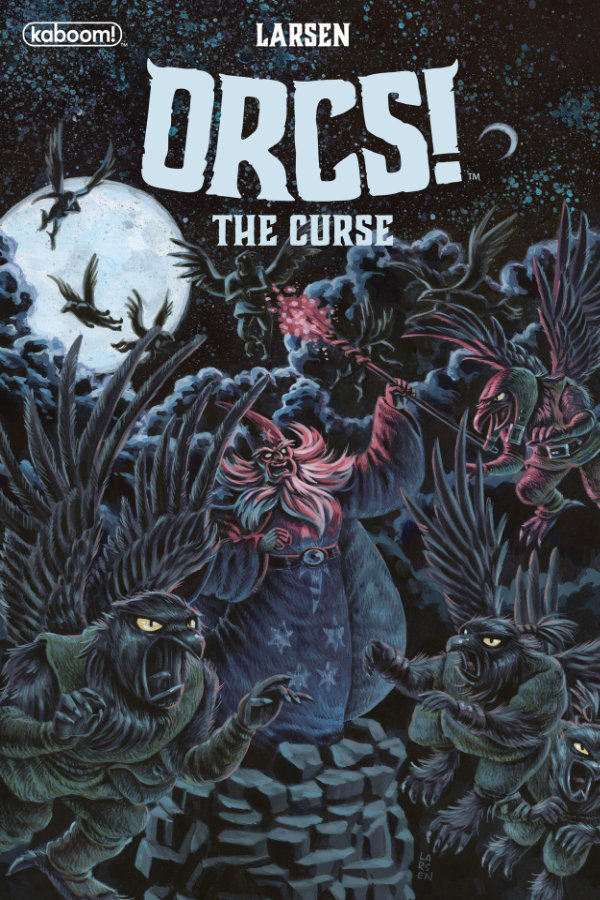The image depicts a highly detailed comic book cover for "Larson Orcs: The Curse" by Kaboom Comics. The Kaboom Comics logo, an oval with lowercase letters and an exclamation point, is located in the upper left corner. At the top center, "LARSON" is written in bold, all caps, followed by "ORCS!" in large, slightly curved letters with a light blue hue. Below this, the subtitle "THE CURSE" appears. The central illustration features a furious wizard with a flowing beard, adorned in a star-pointed hat, wielding a staff emitting flames or sparkles. He stands in a dark forest landscape scattered with gray slate stones and eerie, yellow-eyed creatures lurking among them. The sky is dominated by a full moon surrounded by several dark birds with human-like features, such as bird heads, wings, and clawed human-like hands and feet. To the right of the full moon, a smaller crescent moon and a sprinkling of stars enhance the mystical atmosphere.